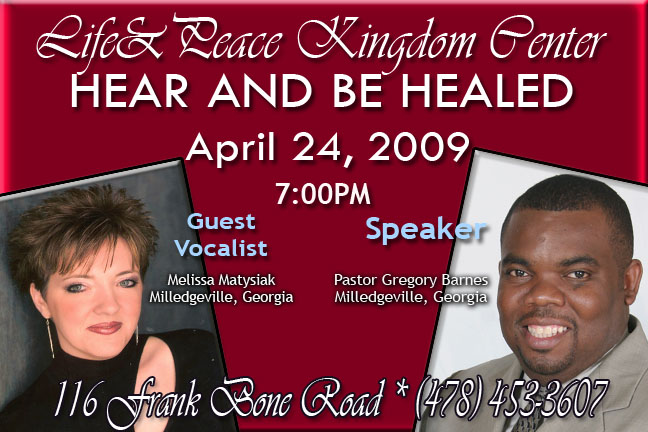This image is an advertisement for an upcoming event at the Life and Peace Kingdom Center. Featuring a red background, the topmost section showcases the center's name in white cursive text. Below that, bold white capital letters proclaim "Hear and Be Healed," followed by the date "April 24, 2009" and the time "7 p.m." In blue text on the left side, it indicates the guest vocalist, Melissa Matysiak, whose photo depicts a stylish white woman with spiky brown hair and a black dress. On the right side, also in blue text, it announces the speaker, Pastor Gregory Barnes, depicted as a smiling black gentleman in a gray suit and tie. Both individuals hail from Milledgeville, Georgia, as noted. At the very bottom, an address in white cursive text reads "116 Frank Bone Road," accompanied by a phone number, "(478) 453-3607."